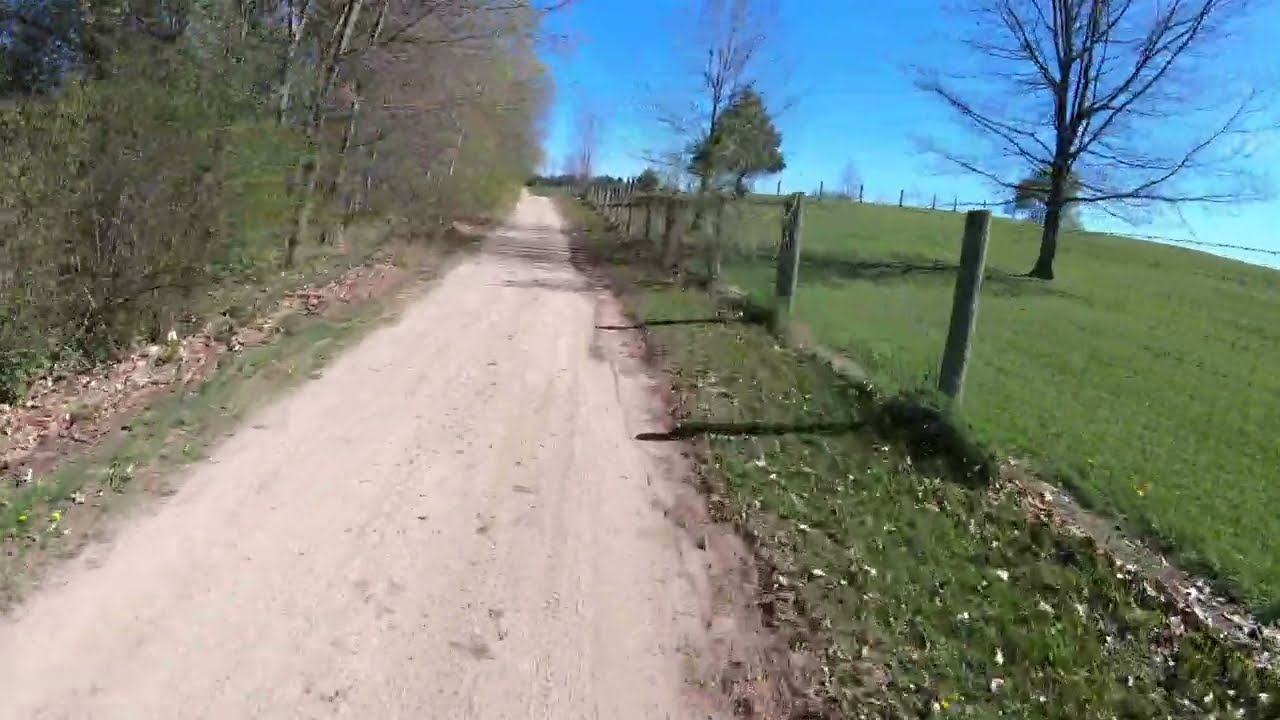The image is a detailed view of a long, unpaved dirt road that stretches into the distance, situated in a rural area during what seems to be an early evening in the fall. The road is flanked by a verdant green lawn on both sides. On the left side of the road, a grove of trees stands tall, devoid of leaves, with scattered green bushes below. Among these trees, there is an evergreen tree that maintains its foliage. To the right of the road lies an open green field, separated from the road by a simple wooden fence with visible posts. This field contains a tree with no leaves near the front and another tree in the distance that still has its full foliage. Between the dirt road and the fence is a narrow strip of grass, suggesting the sparse presence of a possible stream or line of rocks. The background reveals some poles faintly lining the horizon, extending back with the road. Overhead, the sky is a bright blue, adorned with a few white clouds, illuminating the tranquil scene with the gentle light of a low sun.